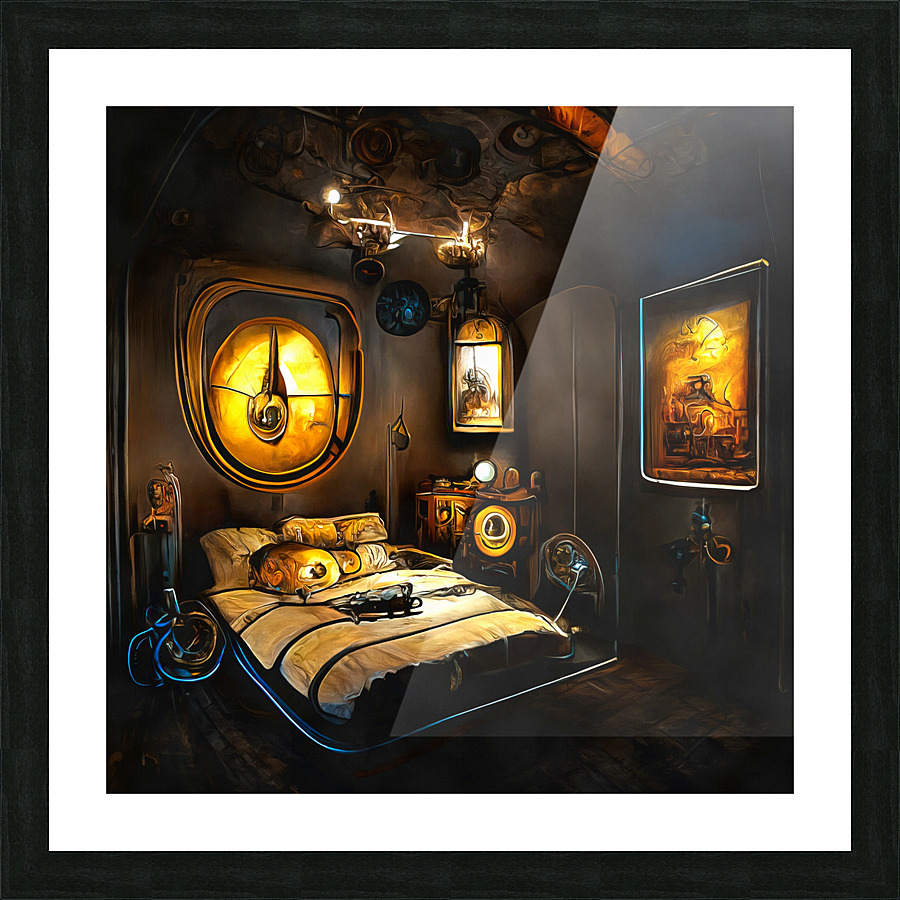This image, which appears to be a detailed and colorful digital painting, is framed in a black border with a white matting. Inside the frame, it depicts an ornate and possibly medieval-themed bedroom with a focus on a bed. The room itself has a curved brown ceiling with a wrinkled texture, and lights are hanging down, illuminating the space with yellow and orange tones. The bed, set at an angle, is covered with a white sheet featuring black stripes and is adorned with various pillows and an indistinct device. To the left of the bed stands a sculpture, adding to the room's decorative elements. Above, candles burn on a circular frame or object, providing a warm glow. There's also a dresser in the corner with a small mirror and assorted items. The room's walls are decorated with pictures and possibly additional lighting. The overall color palette includes black, white, orange, yellow, brown, blue, light blue, red, off-white, tan, and beige, contributing to the image's rich and mystical atmosphere, reminiscent of a scene from an anime.